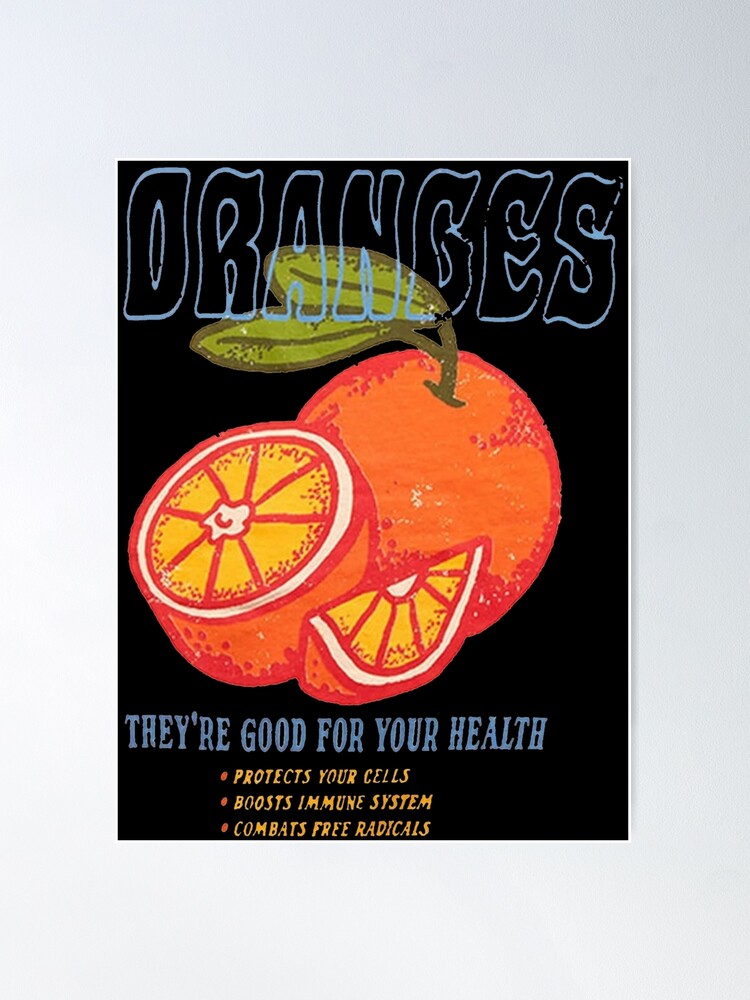This color advertisement, likely for the Florida Orange Growers Association, features a detailed illustration of an orange against a black background. The central focus is a whole orange with a stem and two dark green leaves, alongside a sliced open half of an orange with a wedge, showcasing its juicy, yellowish-orange interior. At the top of the poster, the word "Oranges" is prominently displayed in blue, outlined text. Beneath this, in solid blue letters, it reads "they're good for your health." Further down, three bullet points in yellow text list the health benefits: "protects your cells," "boosts the immune system," and "combats free radicals." The advertisement combines vibrant colors and a clear message to emphasize the nutritional value of oranges.